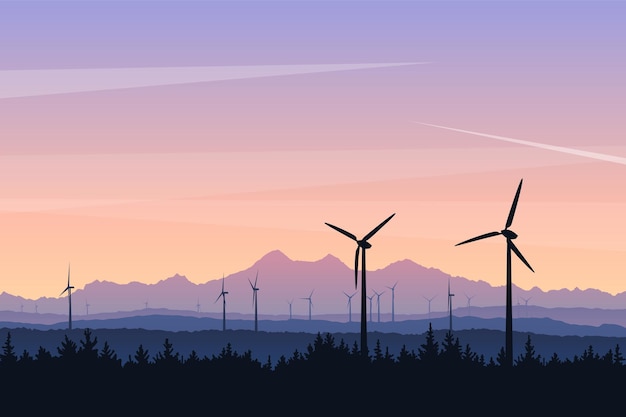This image captures a captivating sunset over a windmill farm, set against a stunning sky transitioning from pastel purple and pink hues to a warm orange. Wisps of white clouds, resembling chemtrails, streak through the sky, enhancing the visual appeal. In the distant background, a lavender-toned mountain range stands majestically. The scene features numerous windmills, their silhouettes blending into the mountainous landscape as they recede into the horizon. In the bottom right foreground, two prominent windmills with three blades each are visible, adding depth to the composition. At the very forefront is a dense tree line, composed of cedar trees, their silhouetted forms framing the lower edge of the image. This serene sunset scene emphasizes the harmony between natural beauty and sustainable energy.